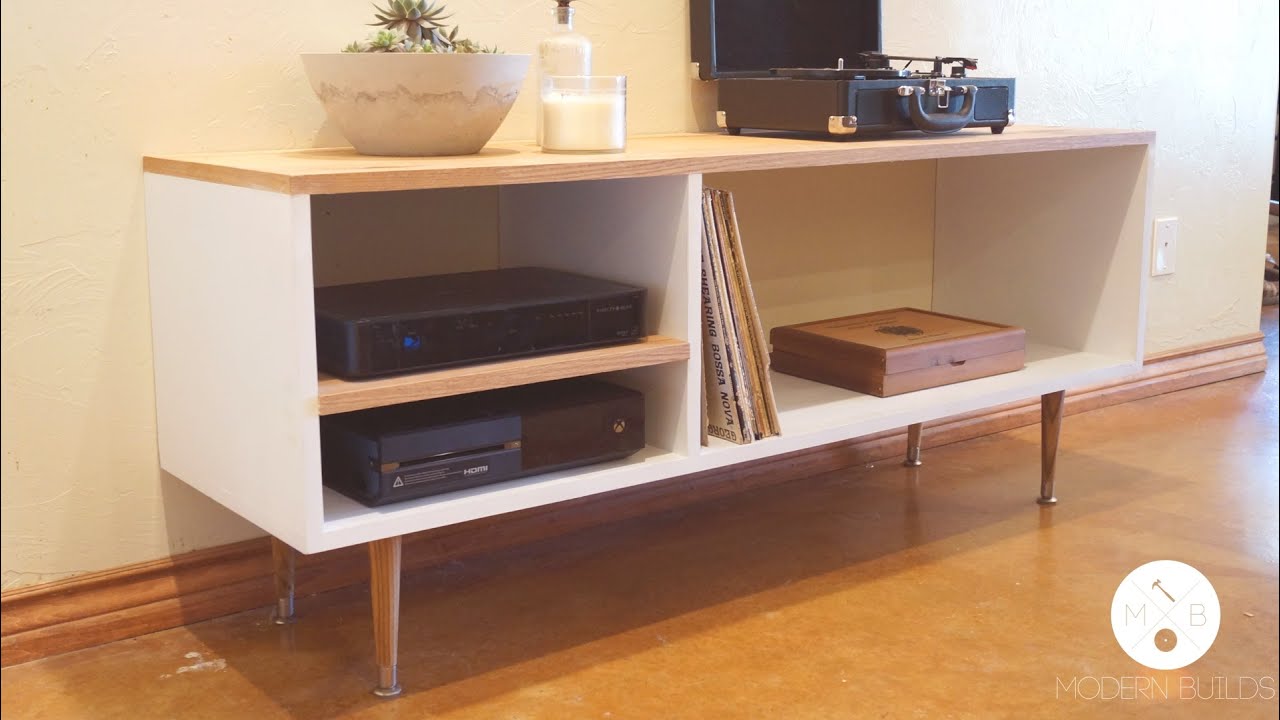Indoor photograph showcasing a meticulously arranged stand against a light tan wall with a brown wood baseboard. The stand, white with four wooden legs and light wood shelves, holds an assortment of items, capturing a blend of modern and vintage elements. The items on the stand include an Xbox One, a candle, a potted plant, a DVD player, and a record player, positioned thoughtfully across the top. Underneath, there are three cubby holes: two on the left housing the DVD player and the Xbox One, and one on the right containing records and a brown wooden case. The floor, light brown with a concrete-like finish, complements the stand while adding a rustic touch to the setting. The photograph is framed with a thin black pinstripe border, and, in the lower right-hand corner, a white circle with a light gray X, featuring a hammer and a brown circle, accompanied by the text "Modern Builds." The dominant colors in the image are blues, blacks, grays, whites, beige, and tan, creating a cohesive and modern aesthetic.